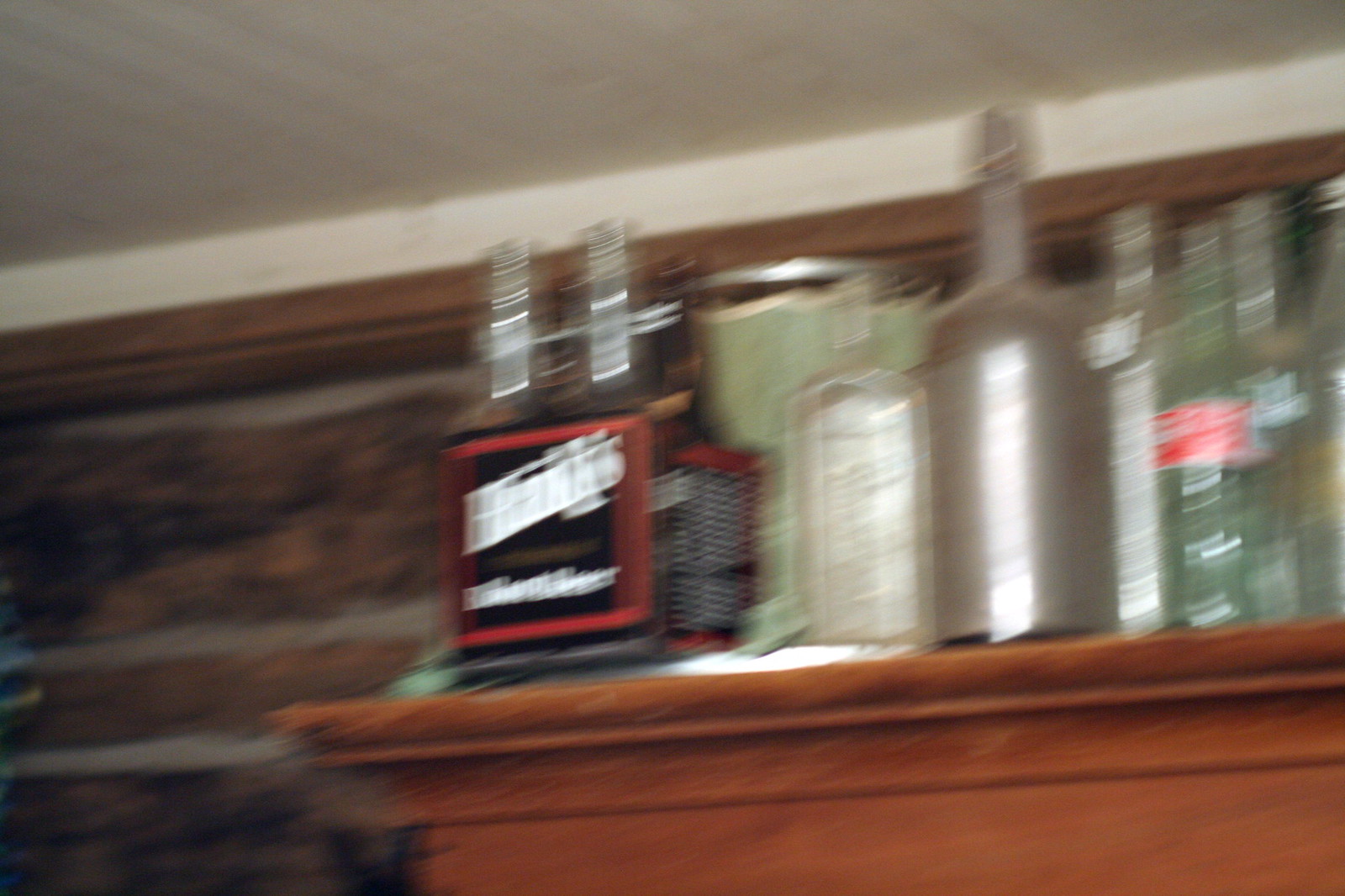This is a blurred image depicting a wooden mantel or tabletop against a brick wall, possibly in an indoor setting like a bar or home. The blurry photograph shows a variety of bottles on the varnished wooden surface, including a distinctive four-pack with red and black packaging and white lettering that likely says "Hank's." There are also clear, mostly empty bottles, with one resembling an older style Coca-Cola bottle. A tall, grayish-silver bottle stands out among them. The scene is captured at a low angle, showing a white ceiling above and a long brick wall in the background. The entire image has a blurred quality, making it difficult to definitively identify all details.